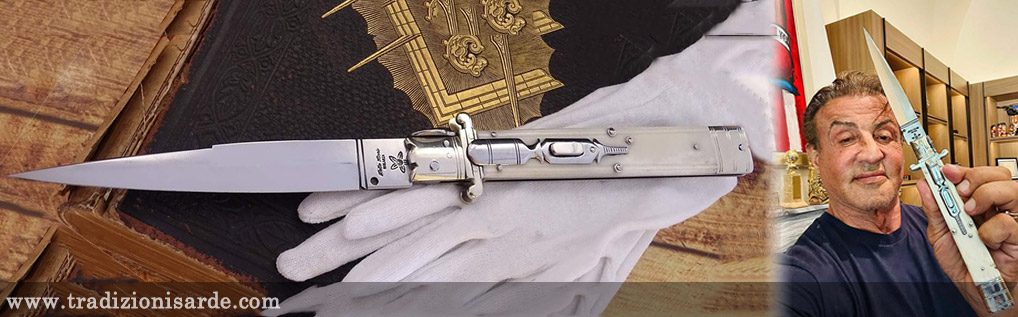The image features a detailed representation of Sylvester Stallone holding a large switchblade knife. The photograph is split into two distinct sections. On the left side, there's a close-up of the knife, which has a blade with a straight line jutting near the center and a decorative element towards the handle. The handle itself includes a small guard on both the top and bottom, along with a white button for extending the blade. The knife is set on a pair of white gloves, with a gold emblem on a black case in the background, all resting on a brown table. A thin black see-through bar extends across this side, and the bottom left corner of the image contains the text "www.tradisarde.com." On the right side of the split, Sylvester Stallone is seen holding the knife upright in his left hand while smiling at the camera. He is wearing a blue t-shirt and is seated in a room with several shelves visible in the background. The image could be a photograph or a highly realistic drawing as it captures Stallone's likeness with great detail, evoking his iconic Rambo persona.